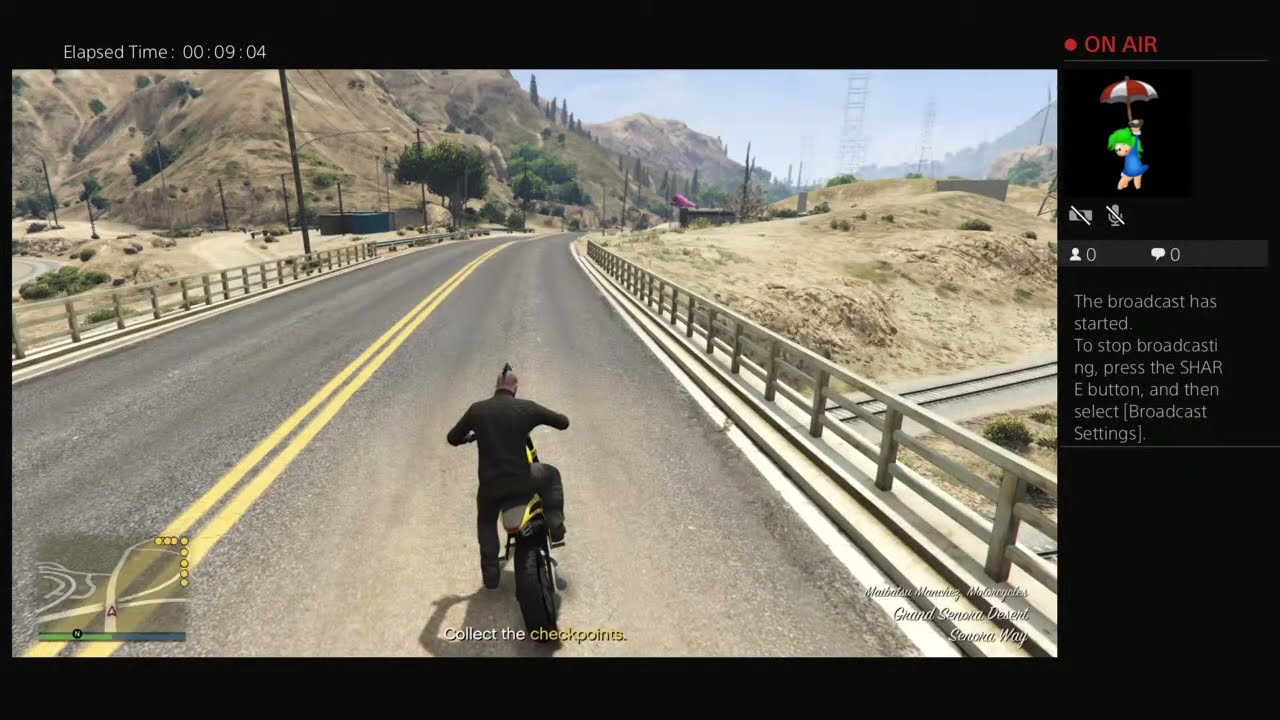In this detailed image, we have a dynamic screenshot taken from a video game, likely akin to Grand Theft Auto. The central focus is on a Caucasian man with a mohawk, dressed in a black long-sleeve shirt and black pants, sitting on a motorcycle positioned at the bottom center of the image. He appears to be paused, with one foot on the motorcycle and the other on the ground, as though he's either just arrived or is about to depart. The single-lane road he's on is flanked by guard rails, suggesting it's a bridge spanning over visible railroad tracks. The surroundings are sandy with sparse vegetation, indicative of a desert-like setting, specifically named the Grand Senora Desert on Senora Way.

The screenshot includes several UI elements indicative of a live broadcast. In the upper header, white text displays the elapsed time of 00:09:04. On the right side, a red dot accompanied by "on air" signifies active broadcasting. Below this, a small figure with green hair, white skin, and a blue outfit holds a red and white striped balloon. There are crossed-out icons for a microphone and camera, indicating inactive audio and video feeds, and text reads, "The broadcast has started. To stop broadcasting press the share button and then select broadcast settings." Beneath is an instruction in yellow to "collect the checkpoints," highlighting the ongoing game objective. The road in front of the protagonist, marked by double yellow stripes, shows a virtual map indicating upcoming curves, enhancing the immersive gaming experience. The palette features diverse colors including black, white, red, green, blue, gray, and yellow, contributing to the vivid and detailed depiction of the scene.